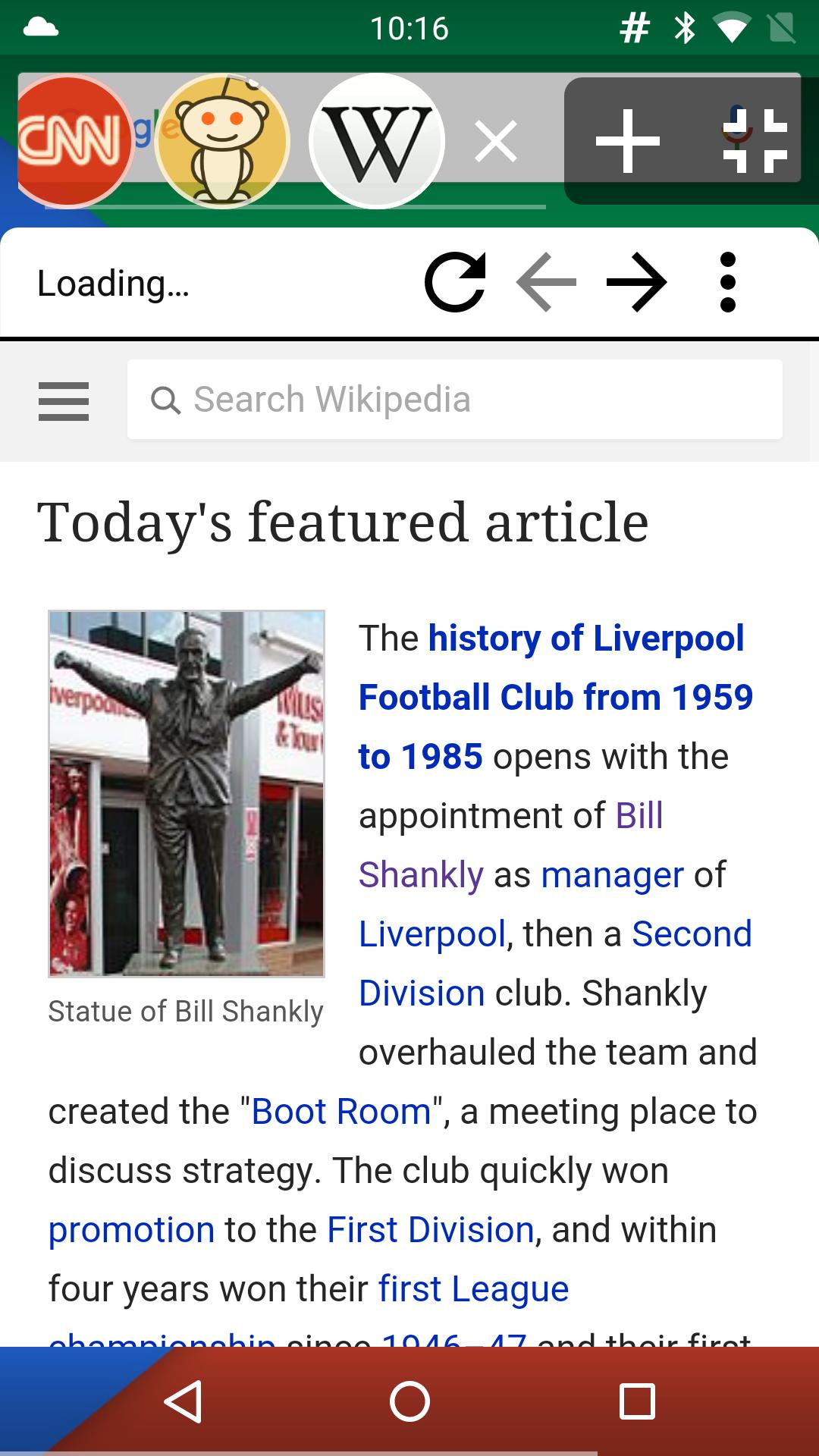A detailed caption for the image could be:

"This image displays a cell phone screen with various elements. At the top, there is a green status bar showing the signal strength, battery life, current time, and a small weather icon. Beneath the green bar, a gray navigation bar contains small circular icons that serve as hyperlinks to different websites. Among these icons are a red one with 'CNN' in white letters, another featuring a white circle with a large capital 'W' indicating a wiki site, and a third icon resembling a small alien figure. 

Further down, the main section of the screen features a white box highlighting a featured article about the history of the Liverpool Football Club. This article includes an image of a statue of Bill Shankly, who is associated with the club's establishment. 

At the bottom of the screen, just below the article, there is a large red rectangle with a subtle blue trim on the edge, which contains page-turn buttons for navigating through the article."